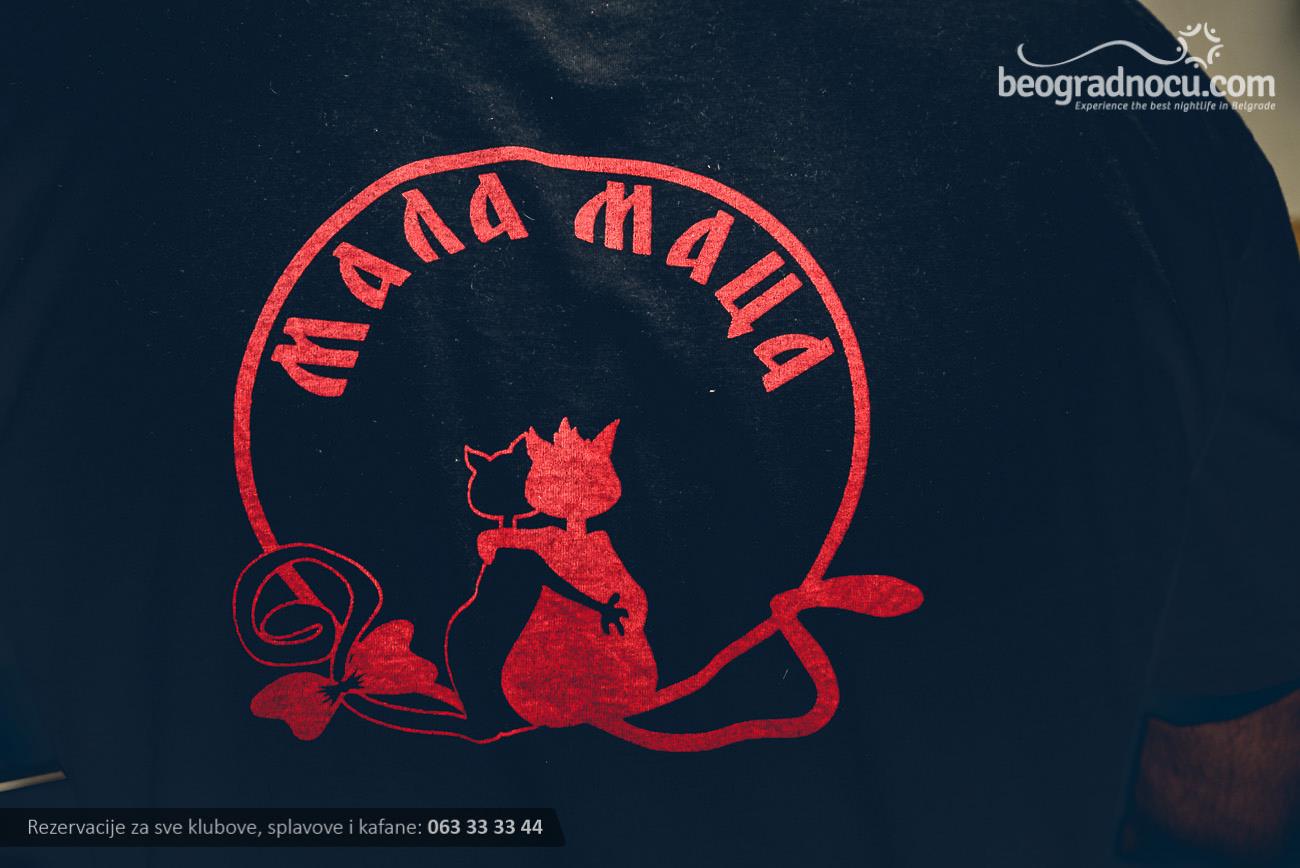The image features a detailed logo on the back of a black t-shirt, worn by a man whose arm is partially visible. The central design of the logo is a red circle containing two cats sitting closely, with their arms around each other in a hugging posture. One cat is red, matching the color of the circle, while the other is black with red outlining. Each cat has a long tail, but the black cat’s tail is adorned with a red ribbon. The circle enclosing the cats bears the words "mana mana." In the upper right corner of the image, there is a watermark that reads "B-E-O-G-R-A-D-N-O-C-U dot com," accompanied by the phrase "experience the best nightlife in Belgrade." Below this watermark, there is additional text in a foreign language and some numbering is noticeable in the lower left corner.